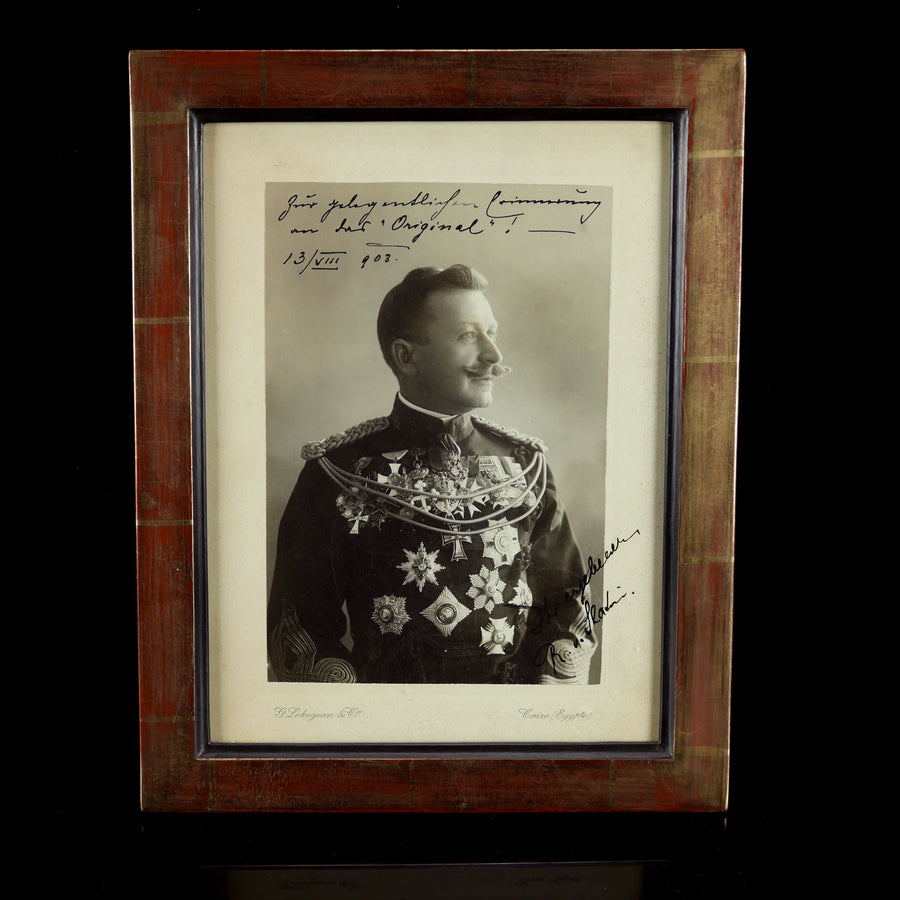This is a detailed photograph of a vintage black-and-white photo, elegantly encased in a thick, dark brown wooden frame with a wide white matte. The central image is an old, black-and-white portrayal of a high-ranking military officer, likely dating back to World War I or II. The officer is looking to the right, his expression calm and composed. He sports a prominent handlebar mustache and has short hair. His uniform is a high-collar jacket, buttoned up to his neck, and adorned with elaborate details. The jacket features ornate patches on both shoulders and is linked by three gold braided ropes running across his chest. His chest and upper stomach are heavily decorated with an array of large metals, including stars and iron stars, signifying his rank and achievements. The photo is further personalized with black ink writing at the top and in the bottom right corner, though the text appears to be in a foreign language and is mostly illegible. The overall presentation, with its historical aura and meticulous details, captures the dignity and distinction of this military gentleman.